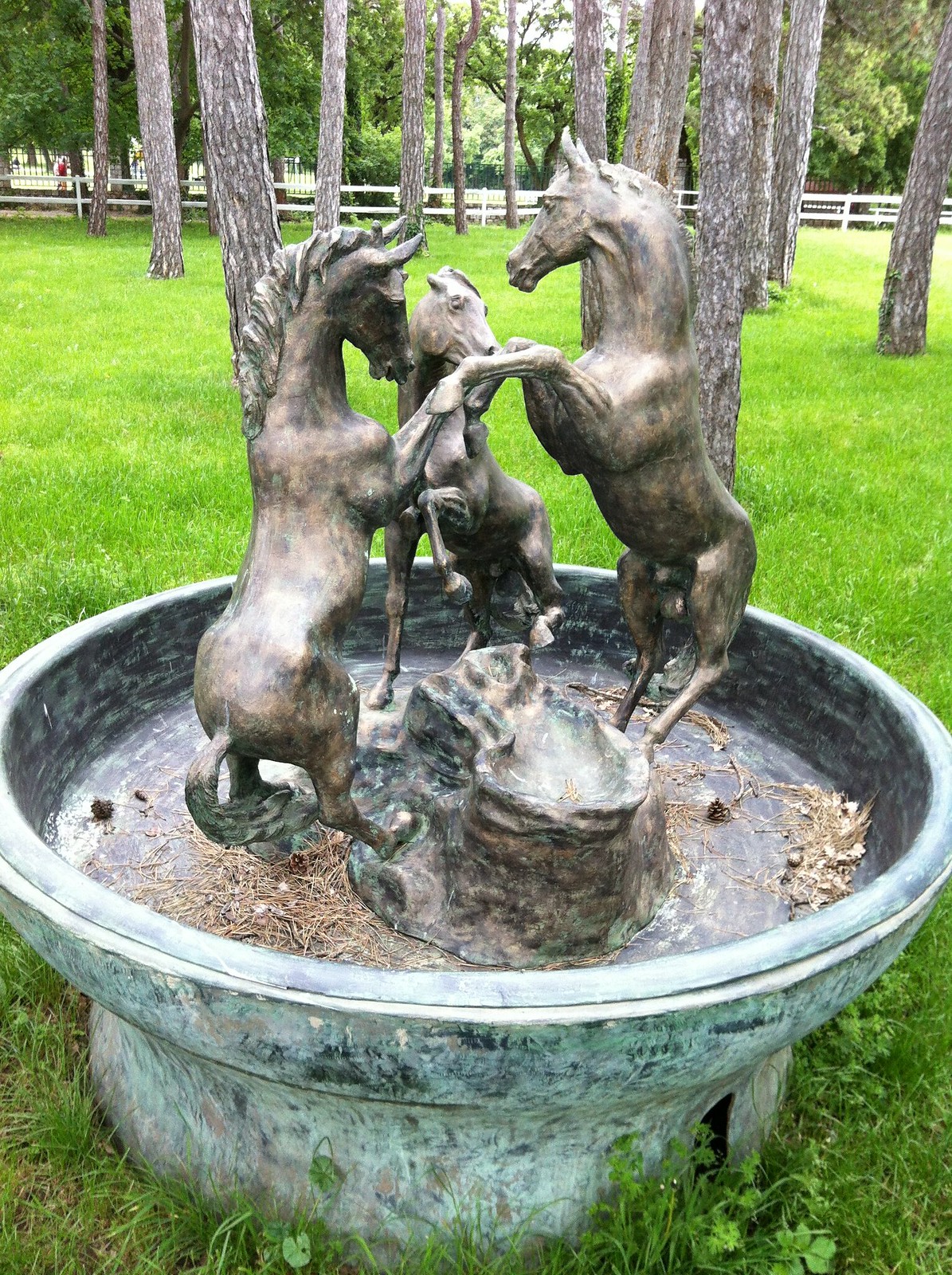This detailed outdoor photograph captures a worn, currently dry stone fountain situated in a grassy park. The fountain, with a large circular base and bowl, is encircled by unmowed green grass amidst an array of slim tree trunks. At the fountain's center is a rocky structure supporting three bronze horses with a bluish patina, arranged as if in dynamic movement. Two of the horses rear up on their hind legs, touching their front legs together, while the third horse has one of its front and rear legs raised, framed against a backdrop of the lush park. The scene also features a short white picket fence composed of two long horizontal boards and regularly spaced posts, behind which more trees are visible. In the far distance, to the top left, a small figure is barely discernible, and a black metal fence runs parallel to the white one. The sky is just peeking through the trees, offering a hint of blue.